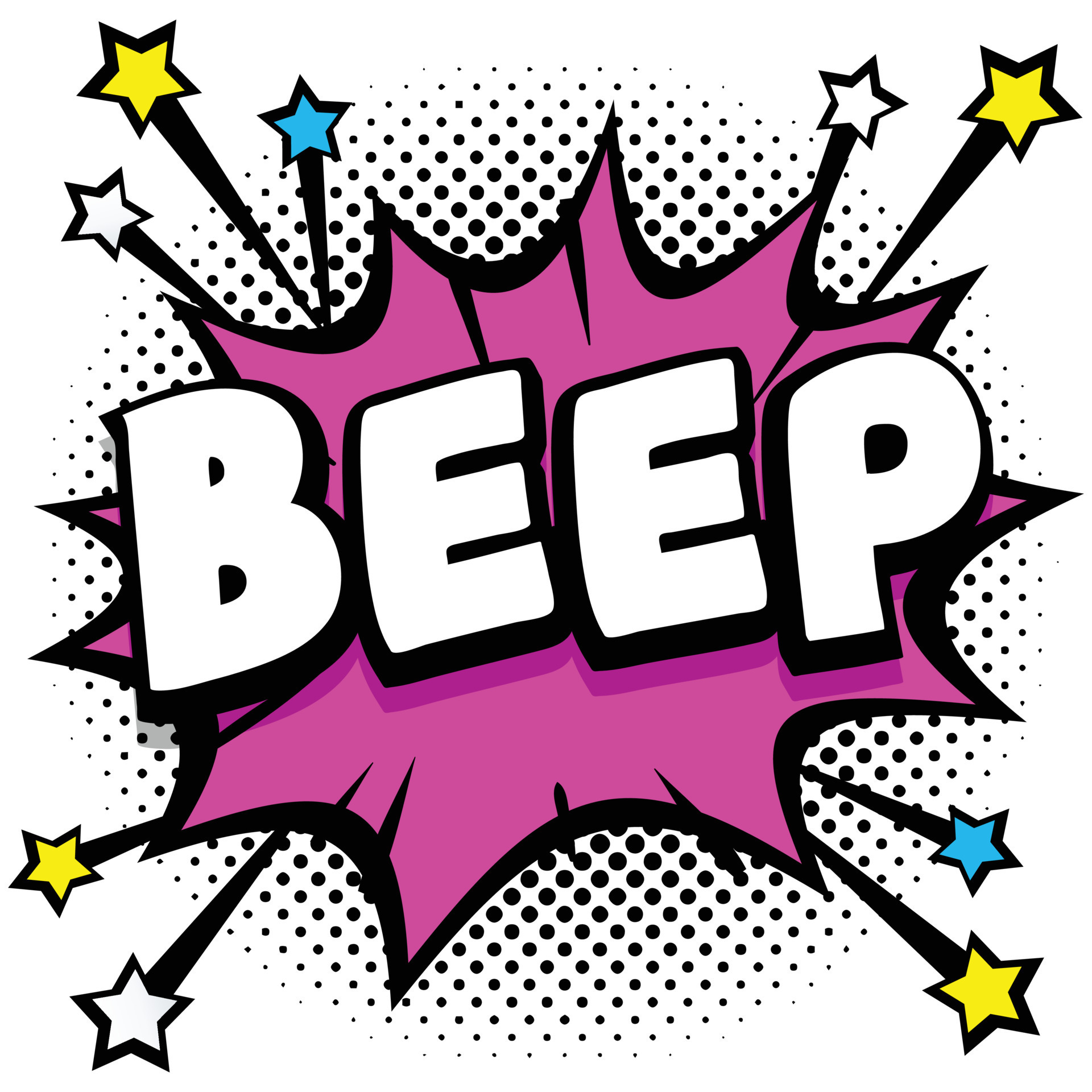This vibrant, comic-style illustration prominently features the onomatopoeia "BEEP" in large, white letters with a bold black outline. The center "BEEP" text is set against a dynamic, jagged starburst shape that resembles an explosive burst, rendered in a rich purple hue with a thick black border. Surrounding the purple burst is a vivid black-and-white polka-dotted background. The black dots radiate outward, starting larger in the center and gradually becoming smaller towards the edges, creating a sense of depth and motion. Additionally, several black lines jut out from the corners of the starburst, adding to the dynamic feel of the image. White, yellow, and light blue stars accentuate the composition, positioned at various points around the burst. The entire scene sits on a clean white background, amplifying the bold and playful aesthetic reminiscent of classic comic book action frames.